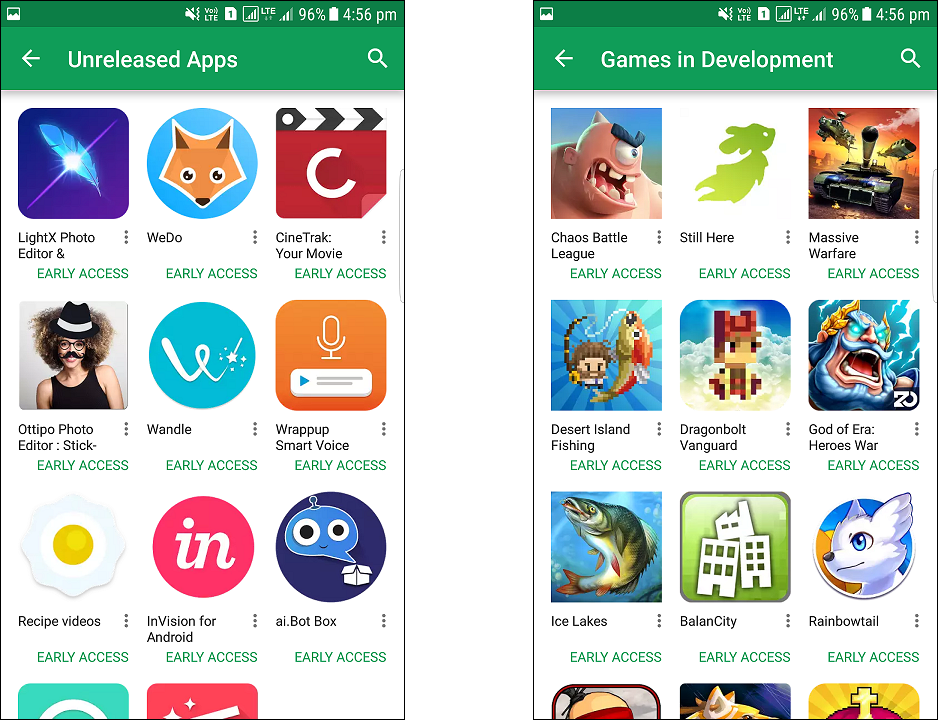This image features two cell phone screenshots side by side. On the left, the screenshot showcases a collection of unreleased apps, while the right side displays games that are in development. Both screenshots have a green status bar at the top, which includes icons such as a mute symbol, reception bar, 96% battery life, and the time, 4:56 PM.

In the left screenshot labeled "Unreleased Apps" in white text, there are nine fully visible app icons arranged in a grid of three across and three down, with two additional icons partially visible at the bottom. The app icons are titled: LightX Photo Editor, We Do, CineTrack Your Movie, Autopo Photo Editor Stick, Wondle, Wrap Up Smart Voice, Recipe Videos, InVision for Android, and AI Bot Box.

The right screenshot, titled "Games in Development" in white text, similarly displays nine fully visible game icons arranged in the same grid format, with three more icons partially visible at the bottom. The game titles include: Chaos, Battle League, Still Here, Massive Warfare, Desert Island Fishing, Dragon Ball Vanguard, and God of Era Heroes War.